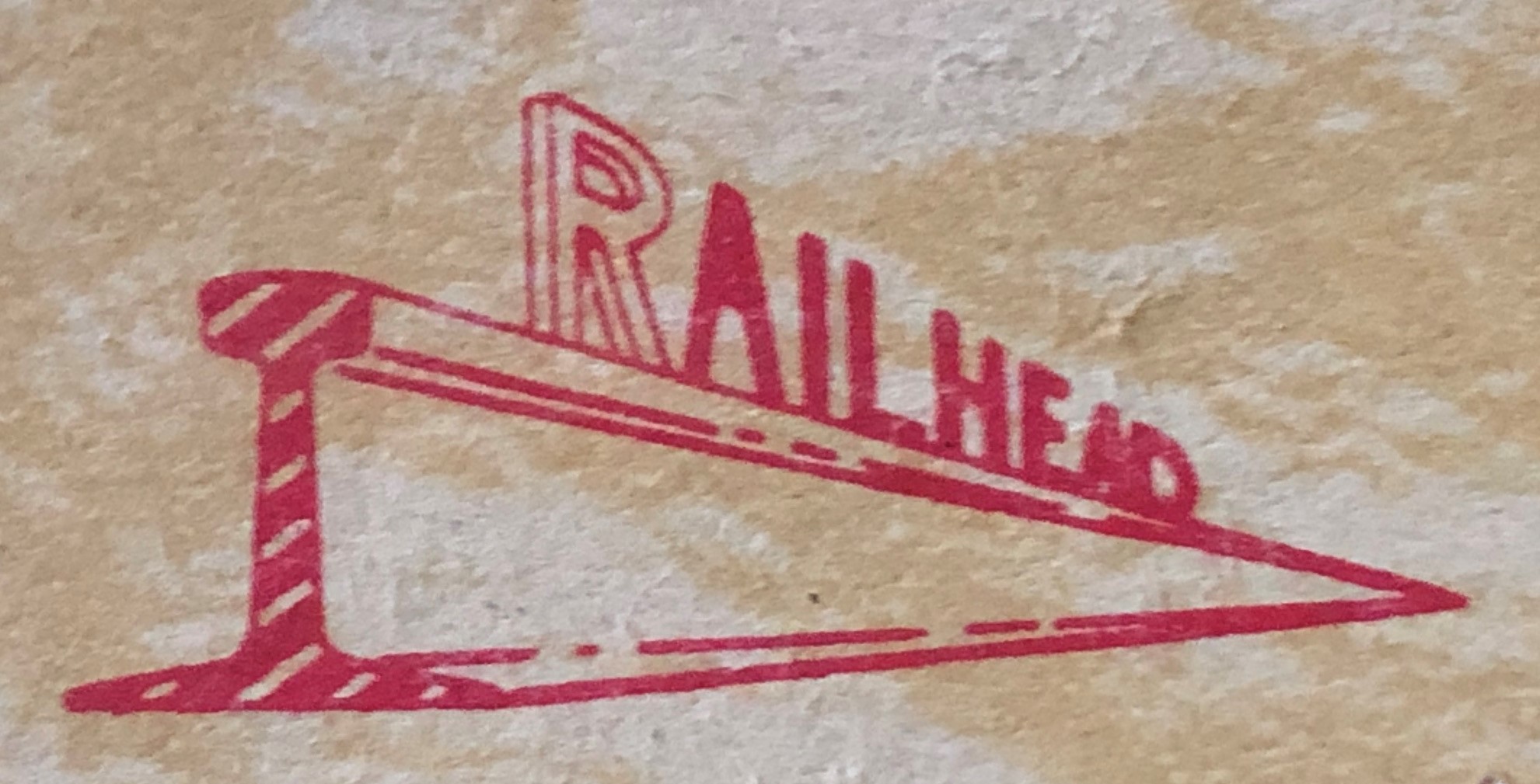The image depicts a closely cropped, zoomed-in photo of Railhead's company logo, stamped onto a surface that might be paper, cardboard, or another fibrous material, though its exact texture is ambiguous. The logo features the word "Railhead" in red capital letters, where the "R" is outlined and three-dimensional, while the rest of the text transitions into a solid red color. The logo includes a stylized representation of a railroad track, rendered in a pinkish-red hue, that tapers into the distance, forming a triangle shape. This track design aligns with the slanted end of the word "Railhead," enhancing the perspective effect. The surface bearing the stamp appears aged, showing varying shades of brown and subtle tears, complementing the vintage aesthetic of the red-stamped logo.